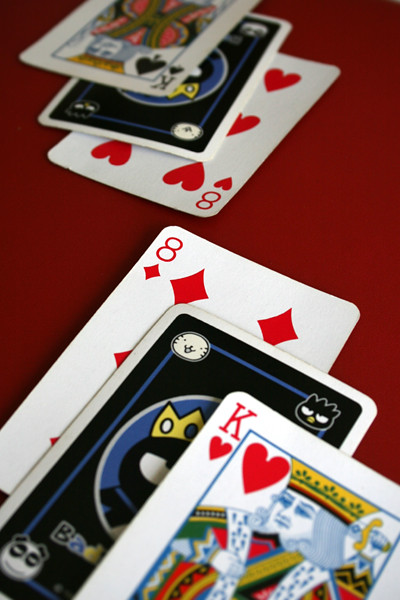In this photo, a smooth red table hosts two neat stacks of cards, positioned on opposite sides of the frame. Each stack contains three cards, with both top cards displaying a king.

On the left side:

1. The topmost card is a King of Hearts. The card features a red heart under the red "K" in the upper left corner, framed by a blue-bordered box showcasing the king's illustration. The king, with blue-toned skin and hairlines, dons a golden crown and an elaborately colored outfit. A red heart is visible next to his face on the left.
2. The middle card reveals the card's back, which is black with a white border. The artwork on the back depicts a cartoon character resembling a duck or a panda situated in the bottom left corner.
3. The bottom card is an Eight of Diamonds, displaying a red "8" in the upper left corner and a pattern of red diamonds down the center of the card.

On the right side:

1. The topmost card is a King of Spades, mirroring the design of the King of Hearts but with spade symbols.
2. The middle card shows another black back with a white border, although the photo does not reveal its specific artwork.
3. The bottom card is an Eight of Hearts, featuring a red "8" in the upper left corner and a pattern of red hearts down the card's center.

The vibrant red table contrasts sharply with the intricate designs and colors of the cards, creating a visually striking arrangement.